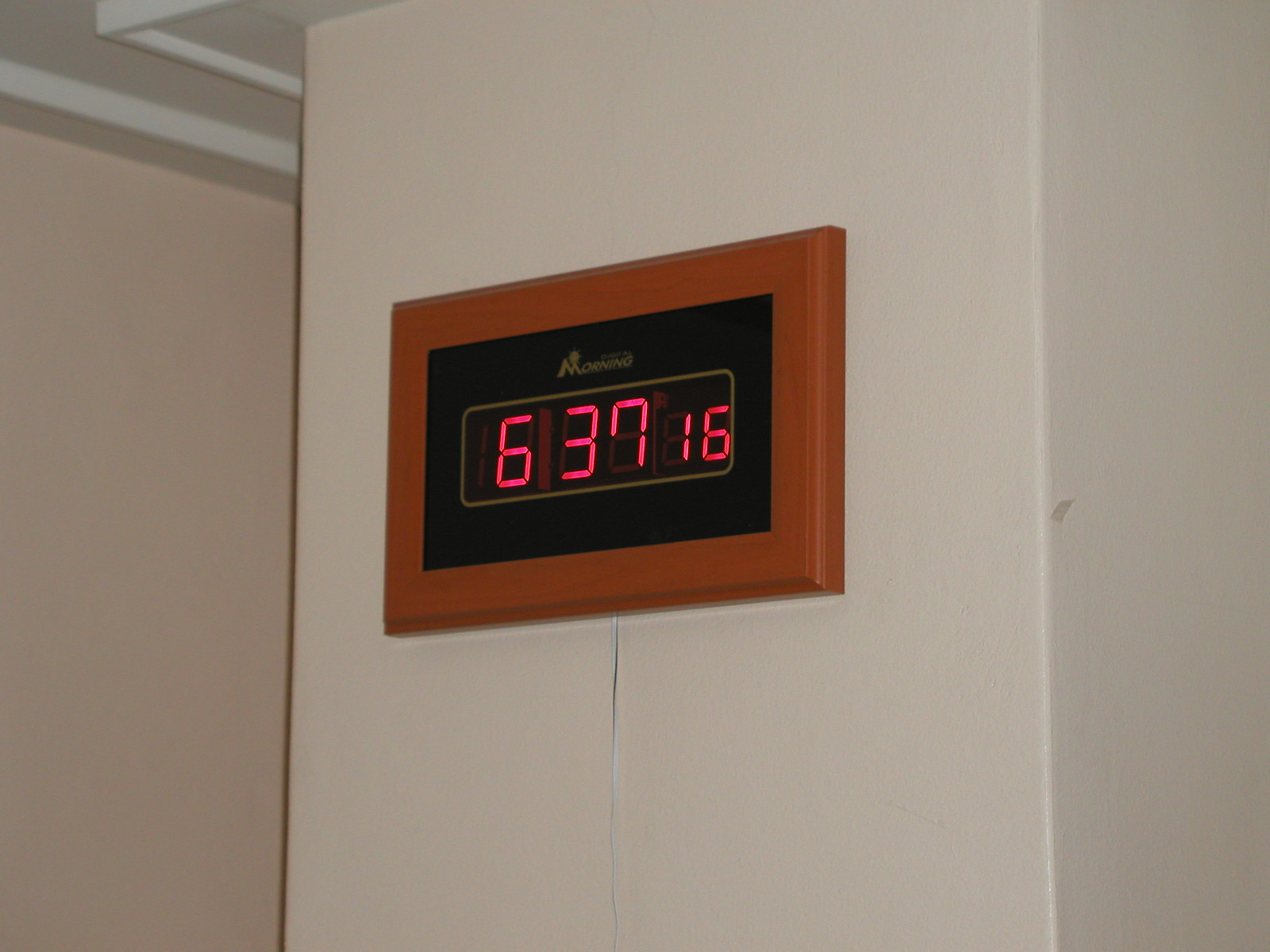The close-up photograph captures a digital clock mounted on a wall, encased in a thick light brown wooden frame. The clock’s display area is black, adorned with white text that may read "Morning" featuring an 'M' topped with a sunrise icon. The time is shown in raised, neon-red digits reading 6:37:16, although there's no indication of AM or PM. A small white border surrounds the LCD screen. The clock is attached to a white-painted wall beam, with adjacent walls appearing white or perhaps cream due to the lighting. Additionally, some close-up details may suggest textural markings and slight color variations on the walls. Above, the ceiling has white paint with some embroidery, and a white cord extends from the bottom of the clock towards an electrical outlet.